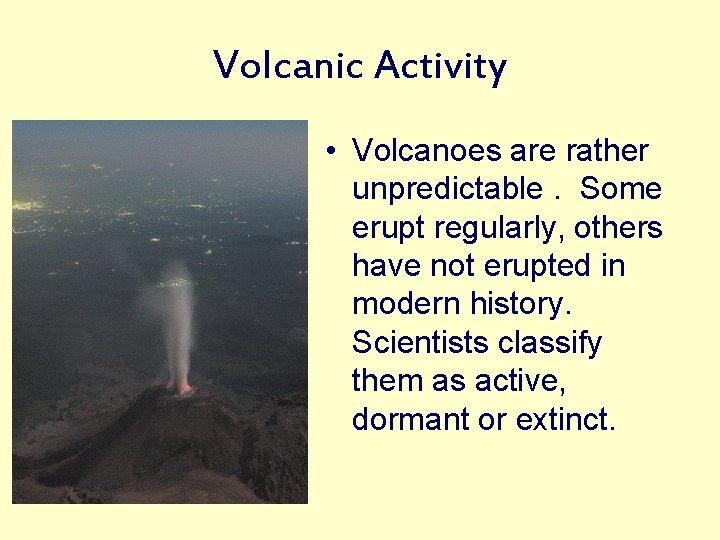The image titled "Volcanic Activity" serves as an informative slide with a light yellow background and blue text. On the left side, it features a detailed picture of a volcano erupting, with a large plume of white smoke and some bright red magma visible at its base. The volcano, appearing brown and steep, stands prominently against a dark sky that melds into the blackness of night. In the background, the image captures a distant city, represented by splotches of tiny white lights, reminiscent of viewing city lights from space.

On the right side of the image, a bullet-point paragraph explains that "Volcanoes are rather unpredictable. Some erupt regularly, others have not erupted in modern history. Scientists classify them as active, dormant, or extinct." The text is positioned next to the volcano picture, reinforcing the connection between the visual and the information presented.

Overall, the image effectively combines visual elements and descriptive text to educate viewers about the unpredictable nature and classification of volcanoes.